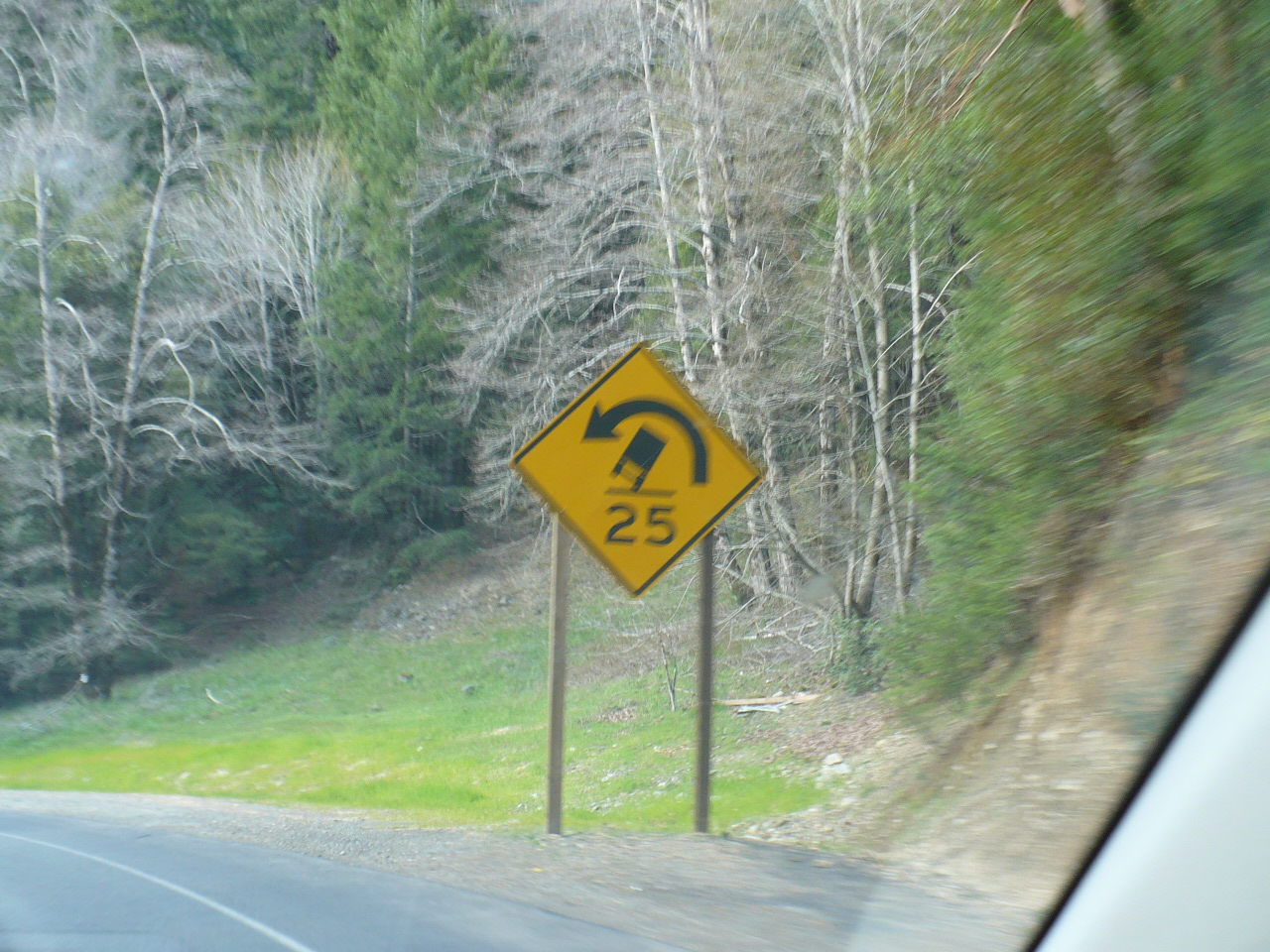The image captures a cautionary road sign as seen through the front window of a car. The scene unfolds on a tree-lined road where slender white birch trees, with sparse leaves, dominate the landscape on the left side of the road. Amidst the greenery of grass and denser foliage in the background, the focal point is a yellow diamond-shaped street sign bordered in black. This sign, mounted on two poles, signals an upcoming curve to the left with a strong advisory to maintain a speed no greater than 25 miles per hour to prevent vehicle rollovers, particularly targeting truck drivers. The road ahead is visible, subtly curving to the left as indicated by the sign, reinforcing the cautionary message.